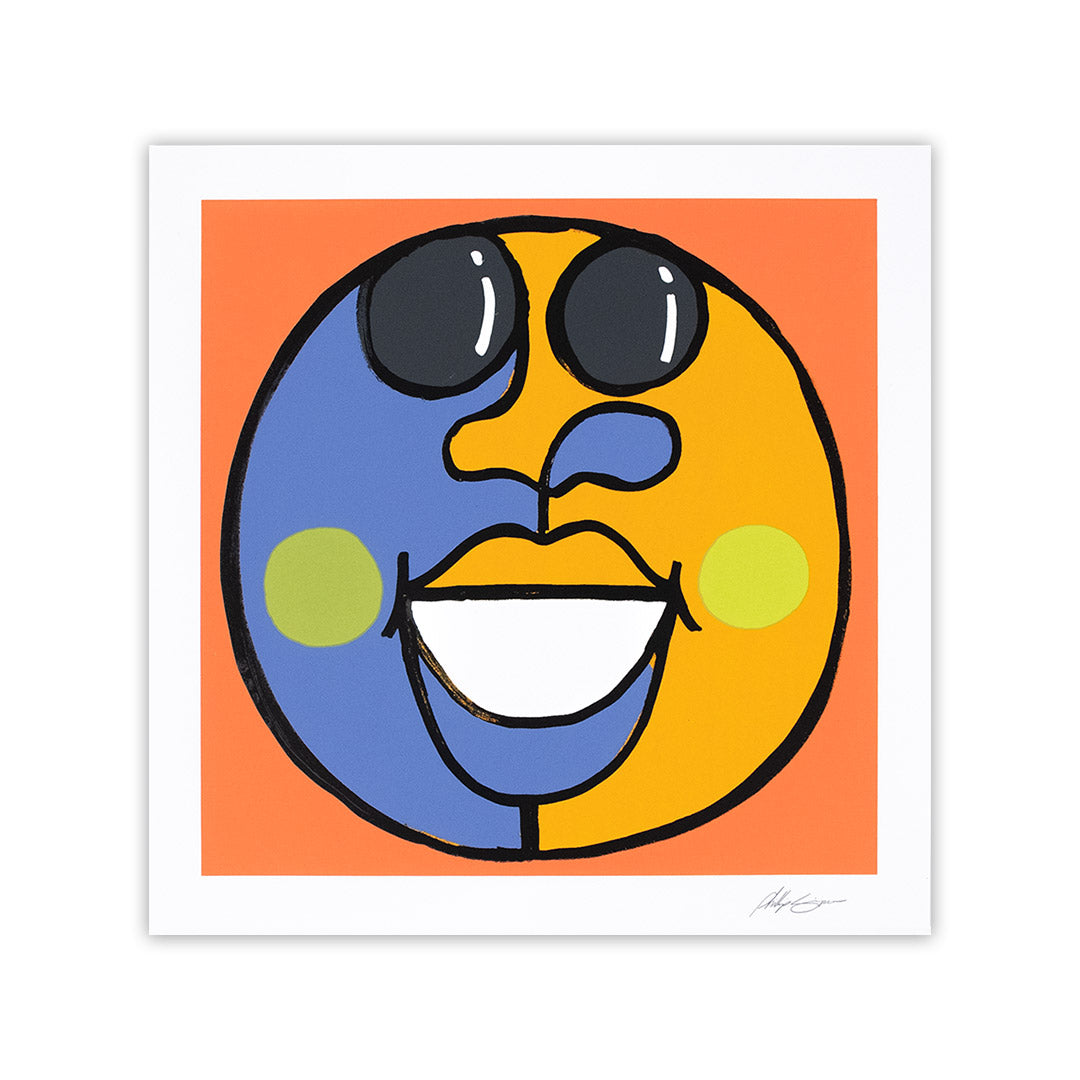The image is a modern art painting featuring a cartoon-like, colorful face with a smile. It is set against a white background with a white square in the center, which has a shadowy black border. Inside this square is a blank white canvas. An orange square placed in the center serves as the background for the face. The face itself is divided down the middle: the left side is blue, and the right side is a yellowish gold. The lips are split, with the upper lip being gold and the lower lip blue, and the inner part of the mouth is solid white. The eyes are two circular dark gray shapes with white highlights. The face also has two muted lime green circles on the cheeks. The nose features a blend of the blue and gold colors, divided down the center, matching the overall color scheme of the face. The style is a blend of op art, modern art, and pop art illustration. A signature in black cursive is present at the bottom right corner of the white matte, but it is illegible.